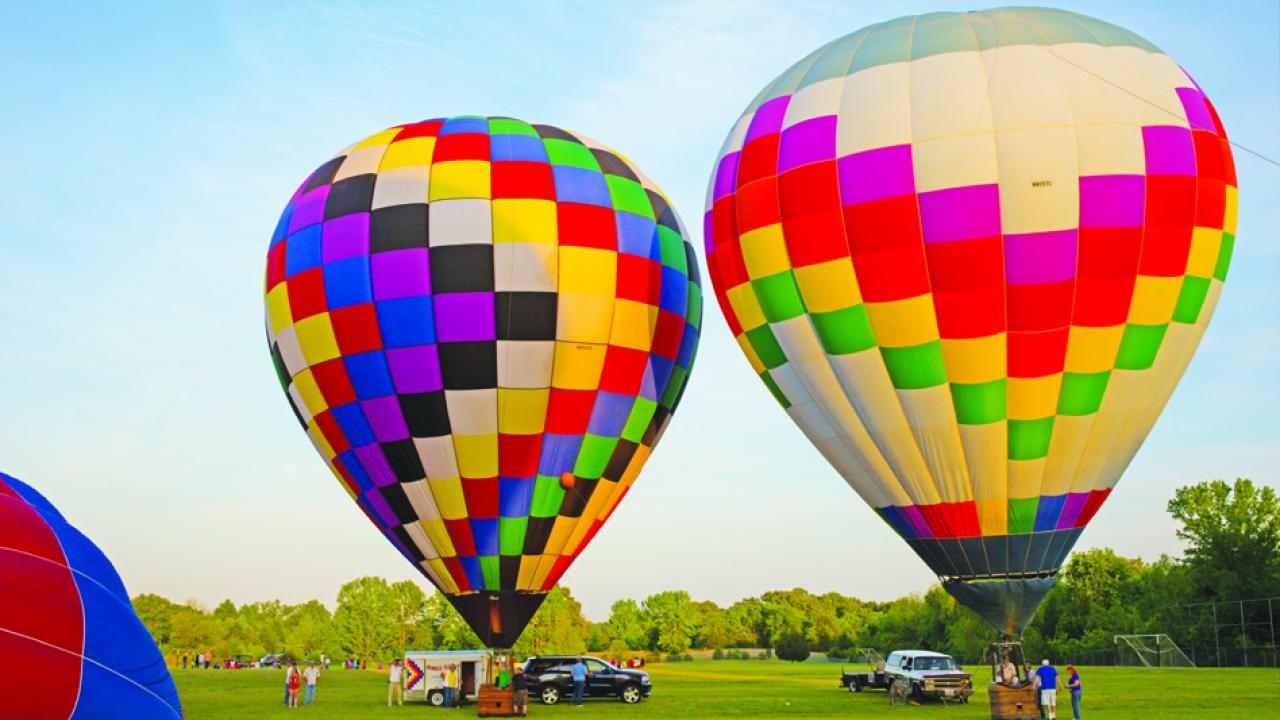The photograph is a rectangular image showcasing an outdoor scene of multiple hot air balloons preparing for takeoff. It captures a large green field, which seems typically used for sporting events, as indicated by a black and white soccer goal with a white net visible in the bottom right corner. The field is surrounded by a scenic line of trees covered with sunlit green leaves, emphasizing the clear blue sky that fades to white near the horizon.

Three hot air balloons dominate the scene. On the bottom left, there is an as-yet uninflated red and blue balloon. In the center of the image stands a fully inflated balloon featuring a patchwork of white, black, purple, blue, red, and yellow squares. Adjacent to it is another colorful balloon with a pattern of blue on top, followed by stripes of white, purple, red, orange, yellow, and green. Both inflated balloons taper down to baskets at their bases, around which people and vehicles, likely used to transport the balloons, are gathered.

Adding life to the photograph, spectators can be seen on the left, watching the preparations, contributing to an overall vibrant and anticipatory atmosphere.